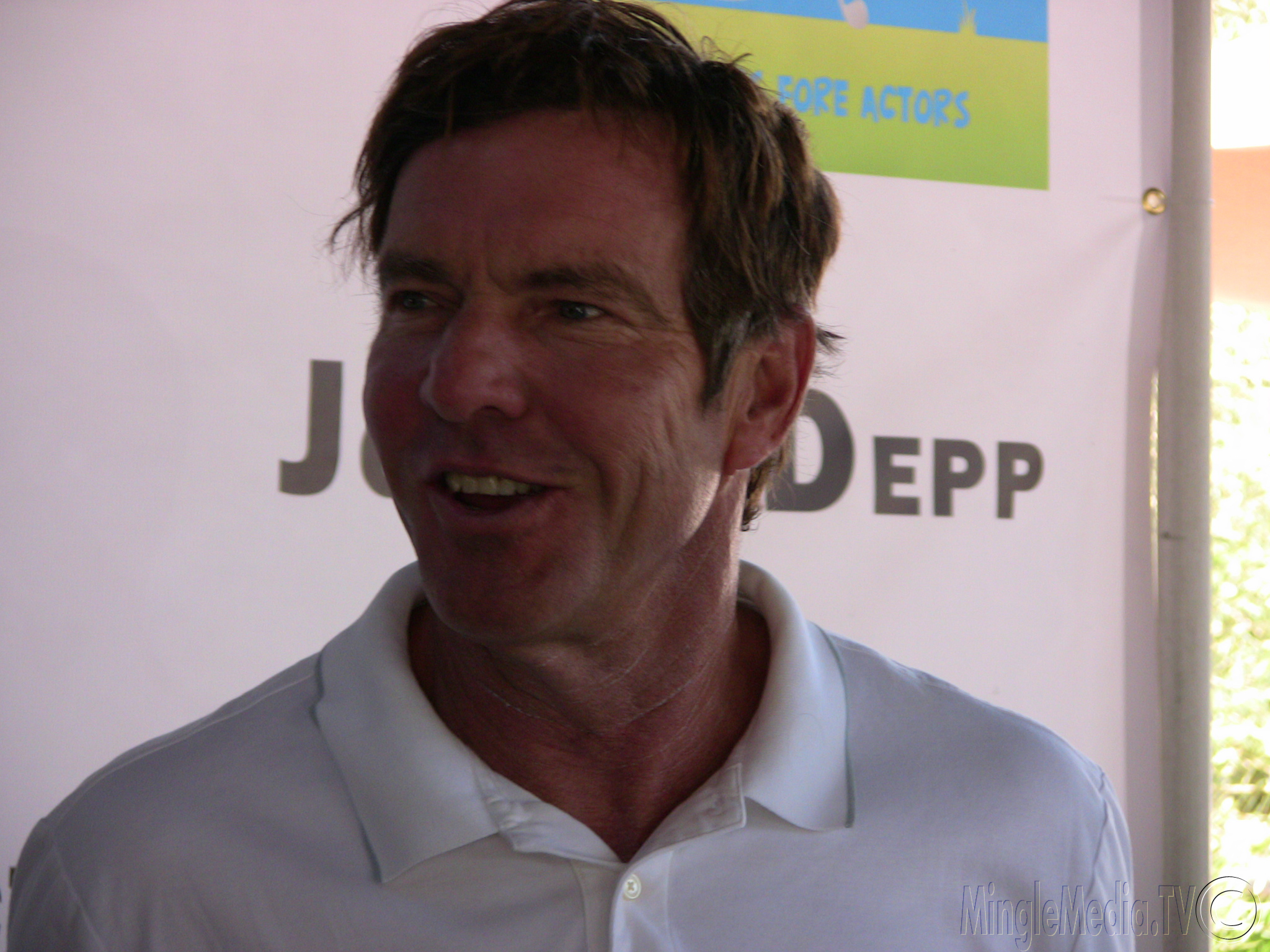In this image, we see actor Dennis Quaid standing outdoors, likely at an actor-related event during the day. Quaid is positioned centrally, wearing a white polo shirt buttoned up to his neck. Behind him is a large, partially obscured white backdrop with the visible text "J" on one side of his head and "DEP" on the other, along with a green square featuring blue lettering that reads "actors." The backdrop prominently displays a watermark stating "Mingle Media TV." On the right side of the image, there are elements of the outdoors including a building edge, grass, and possibly bushes or trees, slightly illuminated by sunlight. The overall color palette includes white, brown, tan, black, green, light blue, and pink, contributing to the detailed and layered composition of the scene.